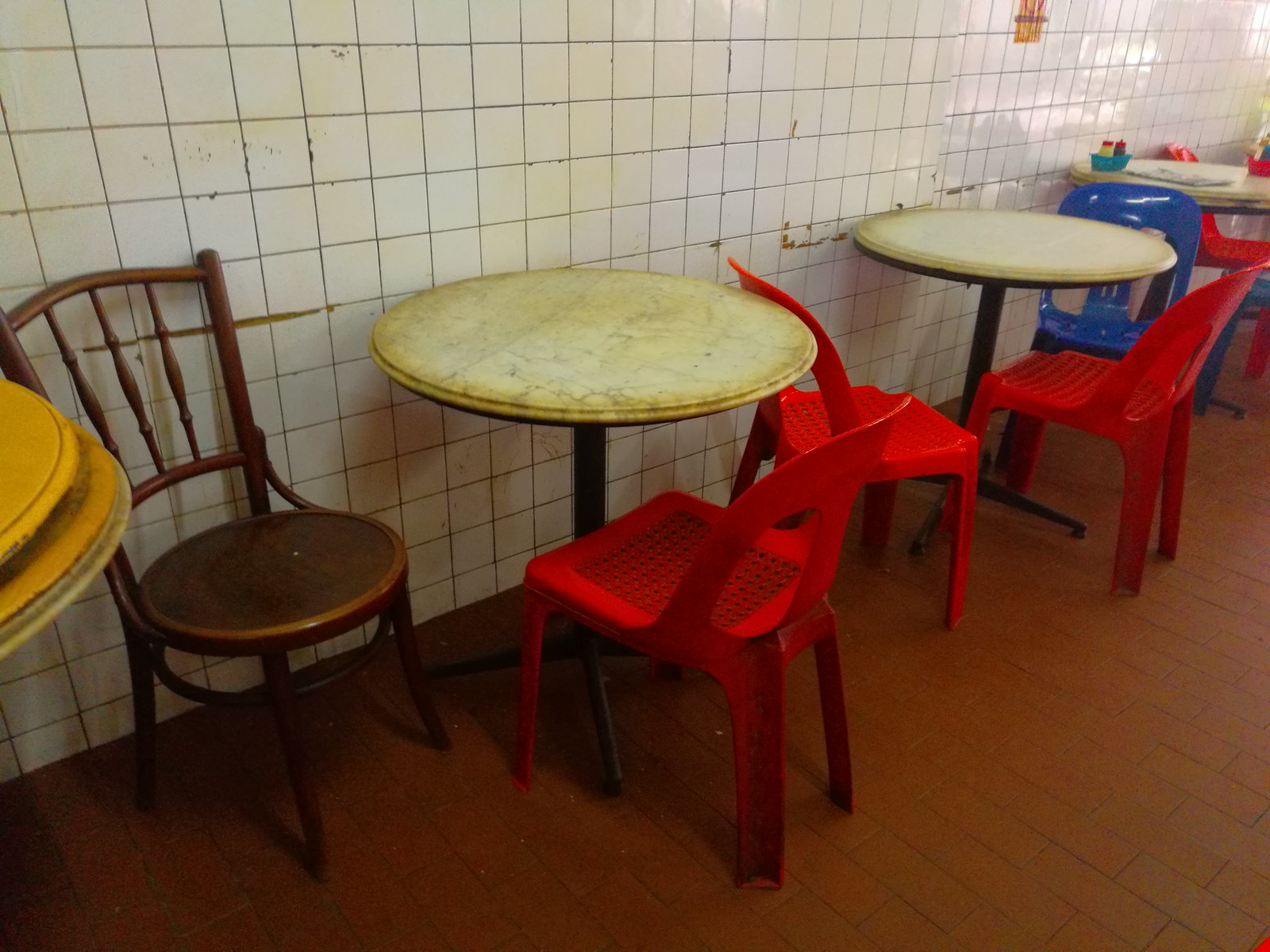The photograph captures a tired and aged small restaurant or cafeteria with a distinct touch of neglect. Dominating the scene, an old, discolored white ceramic tile wall extends from the left to the top right, showing signs of yellowing, scrapes, and dirty patches where the tiles are chipped or misaligned. Along this wall, three small, circular tables are lined up, each with off-white tops standing on black bases with four-legged supports. The tables appear worn and dingy, indicative of a space that hasn't seen use in quite some time. Around the tables, an assortment of chairs is haphazardly arranged: four are red plastic outdoor chairs, two are blue plastic, and one is a wooden dining chair. Adding to the contrast, the floor stands out as relatively new with an inlaid red brick pattern, providing a surprising touch of freshness amid the otherwise run-down ambiance. One of the tables holds scattered papers and a small blue basket containing condiments like ketchup and mustard, hinting at past patron activity. Despite these traces of life, the overall impression of the scene is one of abandonment and desolation.